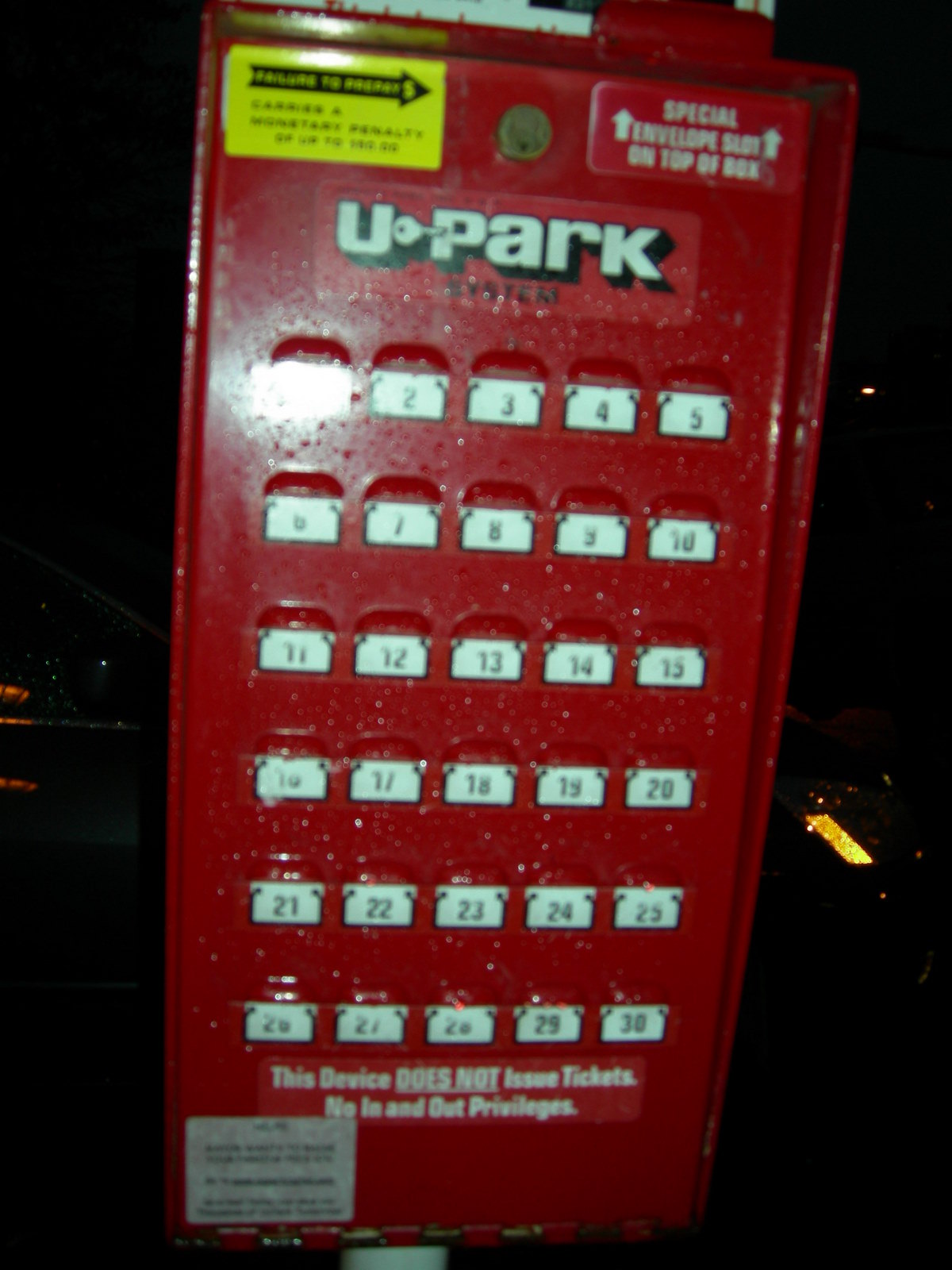The image depicts a tall, rectangular, fire engine red metal machine photographed outdoors at night, as indicated by the black background and the reflected flash partially obscuring the first detail. The top of the machine prominently features a yellow sticker with a black arrow pointing to the right. To the right, there is a red plaque that states "Special envelope slot on top of box," accompanied by directional arrows. Above this plaque is a noticeable brass keyhole.

Beneath these elements, the machine is labeled with the word "Upark," stylized with a letter "U" followed by a key symbol pointing to the right, then the word "Park." Directly under this, "SYSTEM" is printed in black lettering. The machine comprises six rows of numbered white slots, each row containing five slots, labeled sequentially from 1 to 30: the first row ranges from 1 to 5, the second from 6 to 10, continuing in this pattern up to 26 to 30 in the last row.

At the bottom of the machine, additional white text warns users, "This device does not issue tickets, no in and out privileges," serving as an important instruction for its use. This detailed configuration and labeling strongly suggest the machine's purpose is to manage and hold parking lot receipts or keys.